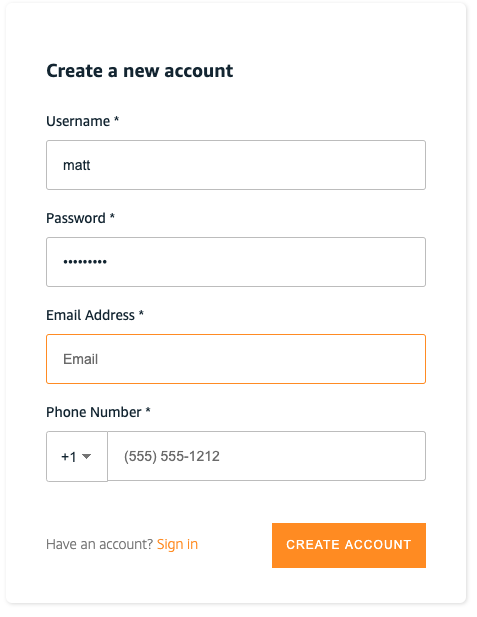The image displays a user interface for creating a new account, potentially from an indeterminate source such as a desktop website, mobile site, or application. The layout lacks identifiable details to ascertain the platform, browser, or device type. Central to the interface is a white box with black, bold text at the top, stating "Create a New Account." The form within the box comprises several required fields, each marked with an asterisk.

- **Username:** Filled in as "matt" in lowercase letters.
- **Password:** Obfuscated with dots, seemingly 8 or 9 characters long.
- **Email Address:** The field is highlighted in yellow and labeled as "email."
- **Phone Number:** Features a dropdown menu for country code selection, currently showing "+1" (the US country code). The phone number entered is a placeholder, "555-555-1212."

At the bottom of the white box, there is a prompt that reads "Have an account?" followed by a clickable text in orange stating "Sign In." Beneath this, an orange rectangular button with white text reads "Create an Account." Although the precise application or website remains unidentified, the form interface clearly serves the purpose of account registration.